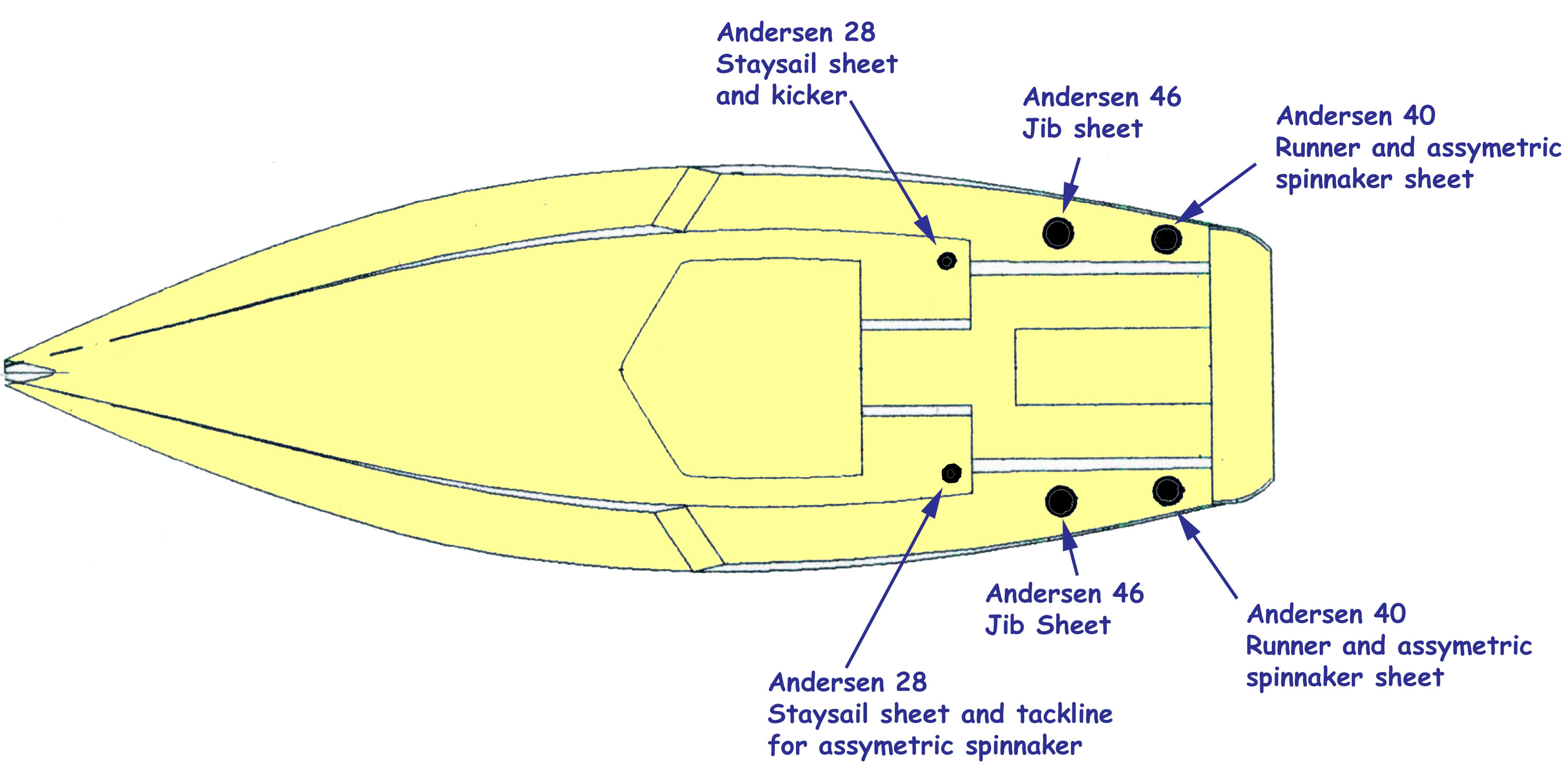The image is a detailed infographic illustrating a top-down view of a speedboat, displayed against a pure white background. The speedboat, reminiscent of a bullet or a soda bottle in shape, features a mostly rectangular back body with curved edges, tapering to a point at the front, which is positioned on the left side of the diagram. The boat is colored yellow.

Numerous arrows emanate from various points on the boat, each accompanied by text explaining specific features. Notably, there are multiple mentions of different components labeled with "Andersen" and numerical designations, implying different functions or parts of the boat's rigging system. These include labels like "Andersen 40 runner and asymmetric spinnaker sheet," "Andersen 28 staysail sheet and kicker," "Andersen 46 jib sheet," and another "Andersen 40 runner and asymmetric spinnaker sheet," highlighting the repetition of certain crucial elements both at the top and bottom of the diagram.